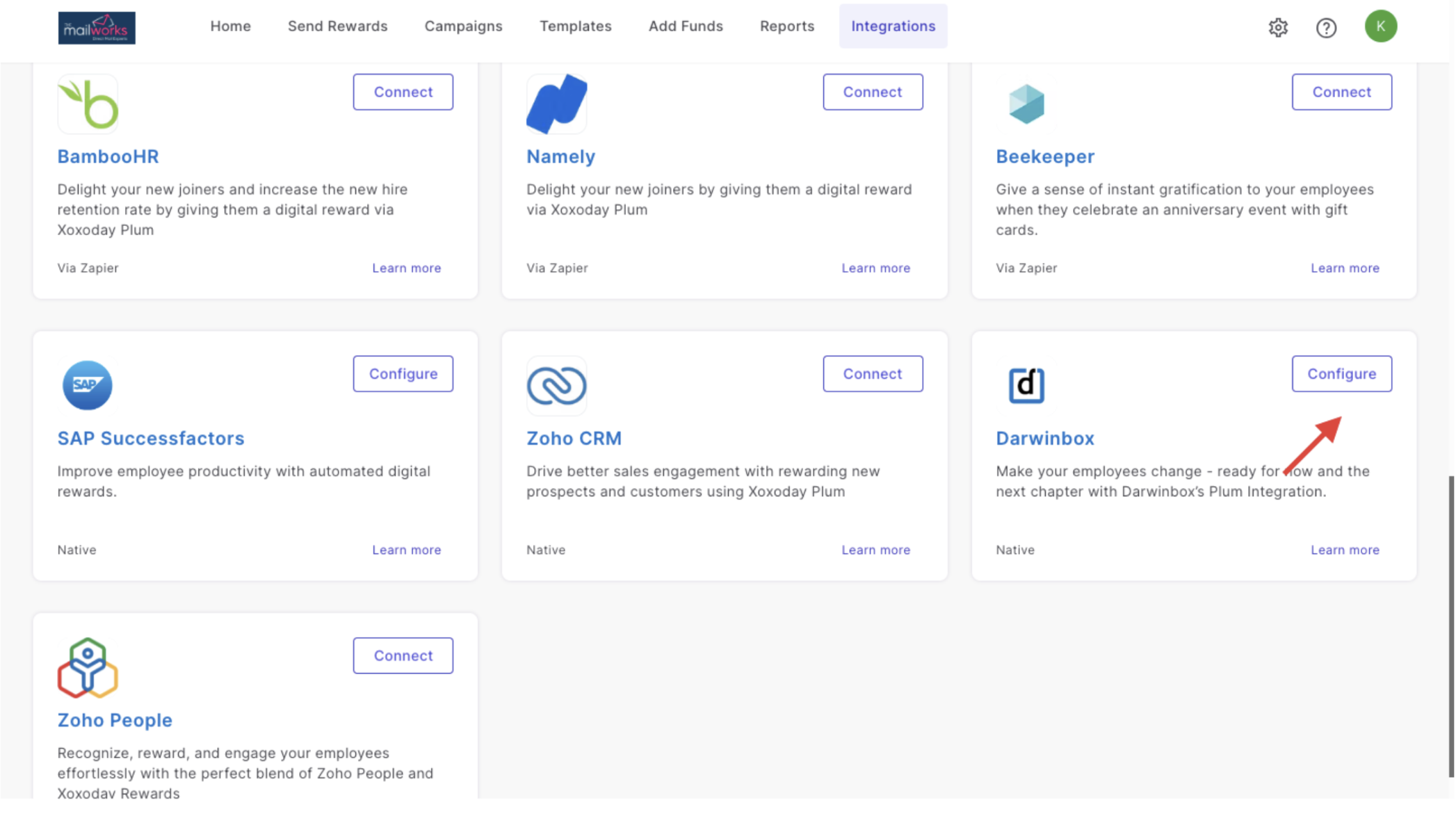The image displays a user interface that closely resembles an app store for business software integrations. At the top left, the partially obscured name "Malworks" is visible. The interface features a navigation bar with sections labeled: Home, Send Rewards, Campaigns, Templates, Add Funds, Reports, and Integrations.

The Integrations section is selected, revealing a grid layout of various business integration options, including Bamboo HR, Namely, Beekeeper, SAP, Zoho CRM, Darwinbox, and Zoho People. Each tile represents a different application that can be integrated into the main platform.

A red arrow highlights the Darwinbox app, accompanied by the text: "Make your employees change-ready for the next chapter with Darwinbox integration." The highlighted Darwinbox app includes a "Configure" button, indicating that the app is already installed and ready for settings customization. The interface overall suggests a focus on enhancing business operations through seamless integration of various software tools.